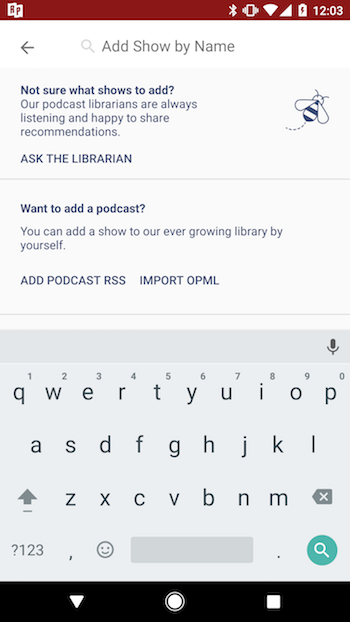This screenshot illustrates a mobile phone application. At the top is a dark red header featuring a white logo on the top left corner, which consists of two slanted rectangles with the letters "P" and "L" in red. On the top right of the header, there are several white icons: a Bluetooth logo, a vibrating phone logo, a Wi-Fi logo, a mobile data icon represented by a triangle, and a battery icon with a red lightning bolt, displaying a time of 12:03.

Below the header, a white navigation bar is displayed with a gray left-pointing arrow and a search bar. The search bar includes a light gray magnifying glass and reads "Add Show by Name." 

The main section contains two separated results with light gray backgrounds divided by a thin gray line. The first result, topped with blue text, reads: "Not sure what shows to add? Our podcast librarians are always listening and happy to share recommendations. ASK THE LIBRARIAN." To the right of this text, there is an icon of a "B" with a dotted line curving to the left.

The second result reads: "Want to add a podcast? You can add a show to our ever-growing library by yourself. ADD PODCAST RSS. IMPORT OPML."

At the bottom of the screen is a QWERTY keyboard, and beneath it, a black footer bar features three white icons: a down-pointing triangle on the left, a circle in the center, and a square with rounded corners on the right.